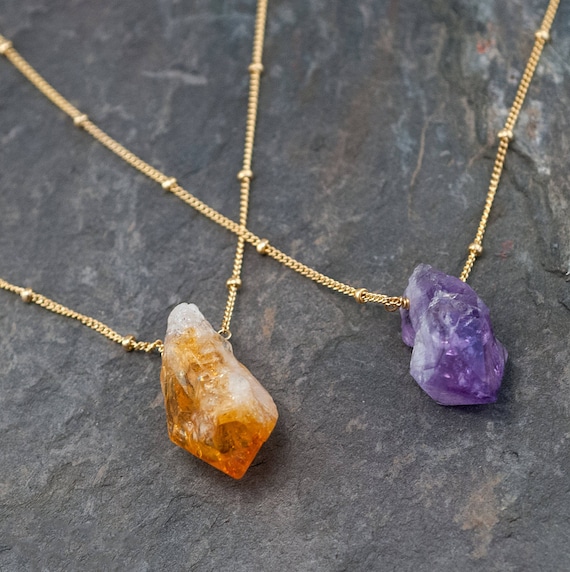In this detailed image, we observe two strikingly natural, unpolished stones positioned on a rugged slate background. The stone on the left is primarily an amber orange with random white streaks cascading across its jagged surface. In contrast, the stone on the right boasts a consistent deep purple hue, also featuring irregular, organic shapes. Both stones serve as pendants, each suspended by gold chains adorned with evenly spaced circular beads, visible only at the bottom of the image where the chains subtly intersect. This close-up view suggests the jewelry pieces are intended as statement accessories, potentially for a necklace or bracelet, alluding to a commercial backdrop for their sale. The entire presentation emphasizes the earthy beauty and natural irregularity of the stones against the textured gray slate, devoid of additional text or visual distractions.